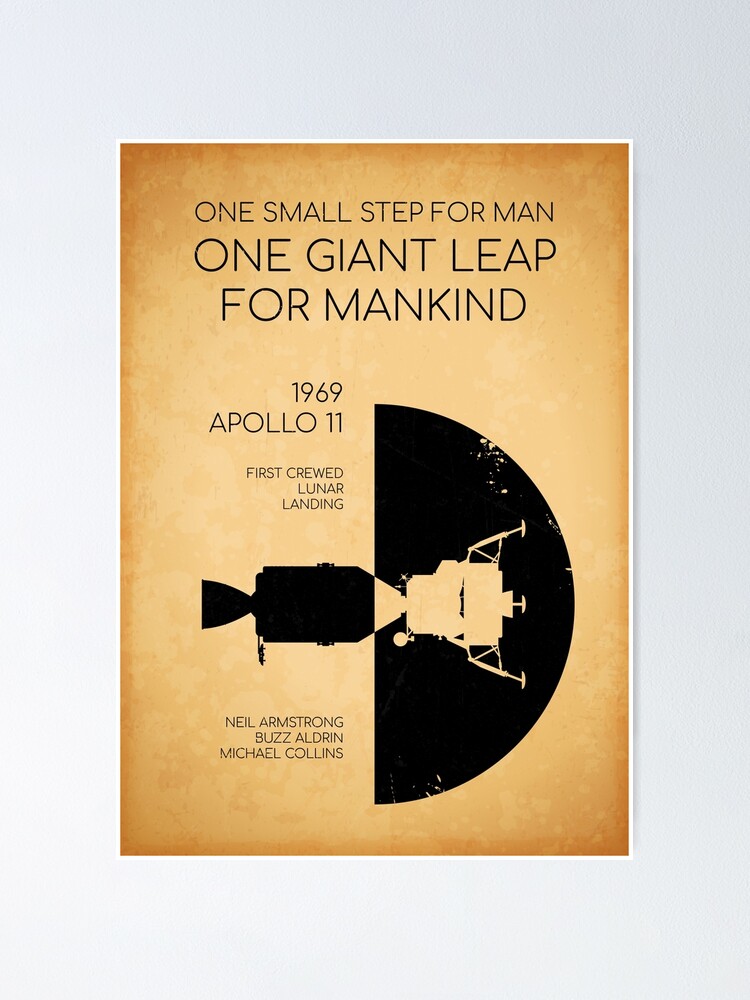The poster, with a portrait layout, features a vintage aesthetic owing to its aged, brownish-tan background that fades from darker edges to a lighter center, bordered by a thin white line. The background outside the poster is a subtle grayish off-white. At the top, in bold uppercase black letters, the famous quote "ONE SMALL STEP FOR MAN, ONE GIANT LEAP FOR MANKIND" is prominently displayed over three lines. Below this, the text reads, "1969, APOLLO 11, FIRST CREWED LUNAR LANDING." Central to the poster is a black and white abstract illustration depicting the lunar module partially overlaid on a half-circle representation of the moon’s dark surface, giving an eerie, dramatic effect. At the bottom left corner, the names of the historic astronauts—Neil Armstrong, Buzz Aldrin, and Michael Collins—are listed in succession.